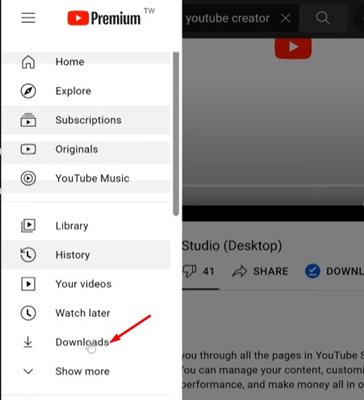The image showcases the YouTube Premium interface with an emphasis on its sliding menu. The menu is extended from the right side of the screen, partially obscuring the background video, which appears to be a tutorial on managing YouTube content and navigating YouTube's pages. The prominent YouTube logo—a red rectangle with a play arrow—is displayed, accompanied by the "Premium" label, signifying the subscription status.

At the top, a hamburger menu icon is visible, followed by several navigation options: a house icon labeled "Home," a compass icon for "Explore," and stacked boxes with a play button signifying "Subscriptions." Additionally, there's an option labeled "Original" with a play button, a target icon for "YouTube Music," a library icon, a clock with a counterclockwise arrow for "History," an arrow in a box for "Your Videos," a small clock for "Watch Later," and a downward-facing arrow indicating "Downloads." Below these, an option labeled "Show More" suggests further menu items not fully visible in the current view.

A red arrow has been added to highlight the download options within the menu. A scroll bar on the right hints at additional content accessible through scrolling.